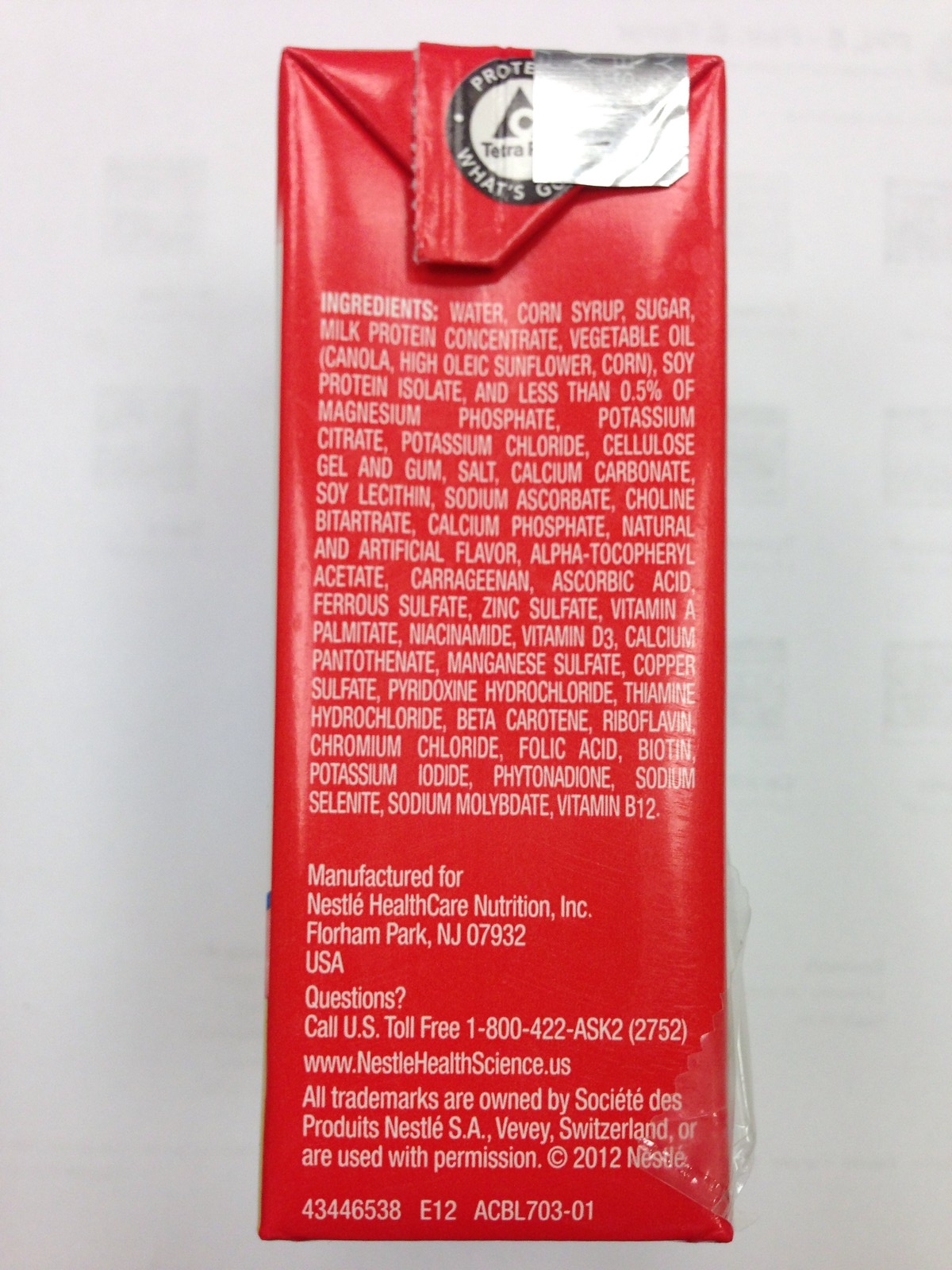This photo features a red, thick, square paper container with a silver top, typically used for products like broth. The side of the container lists the complete ingredients of the food product inside, including water, corn syrup, sugar, milk protein concentrate, various vegetable oils (canola, high oleic sunflower, corn), soy protein isolate, magnesium phosphate, potassium citrate, potassium chloride, cellulose gel and gum, salt, calcium carbonate, and less than 0.5% of soy lecithin. At the top of this list, the word "protein" is prominently displayed. Below the ingredients, it states that the product is manufactured for Nestle Healthcare Nutrition Incorporated, based in Floorham Park, New Jersey, 07932, USA. For inquiries, there's a US toll-free number 1-800-422-2752 and a website www.NestleHealthScience.us. It also mentions that all trademarks are owned by Societé des Produits Nestlé, S.A., Vevey, Switzerland, or are used with permission, copyrighted in 2012 by Nestlé. The package is set against a white background and includes a gray background behind the text, along with a series of numbers: 43446538E12ACBL703-01.